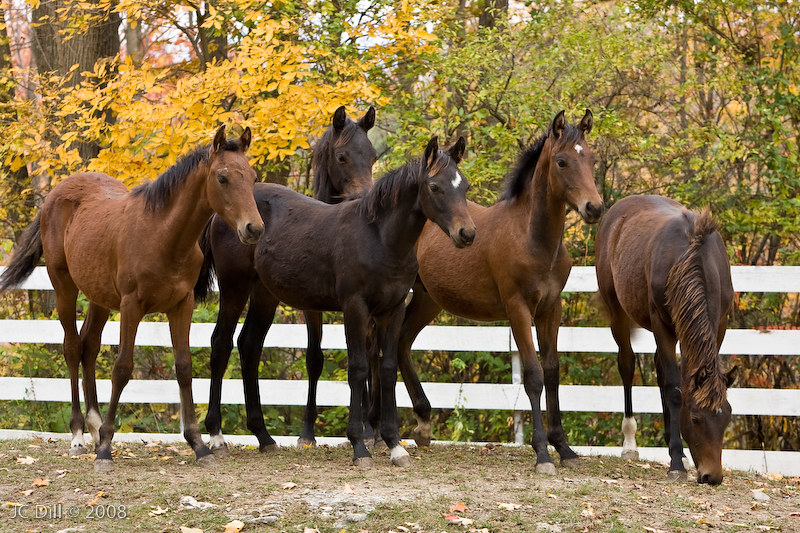This landscape photograph, credited to J.C. Dill in 2008, captures an autumnal paddock scene outlined by a white, three-board slat fence. Set against a backdrop of tall trees with wide trunks and a mix of vibrant green, golden yellow, and some red leaves—indicators of fall—the ground is a blend of dirt, rocks, and sparse dry grass. Inside the fence stand five young horses, their coats ranging from various shades of brown to red. Two of the horses feature distinctive white patches on their foreheads. The horses appear to be yearlings, all standing together and mostly gazing towards the right, except for one red horse on the far right, which is grazing with its head down. The peaceful scene is punctuated by the watermark in the lower left corner that reads "JC Dill Copyright 2008."